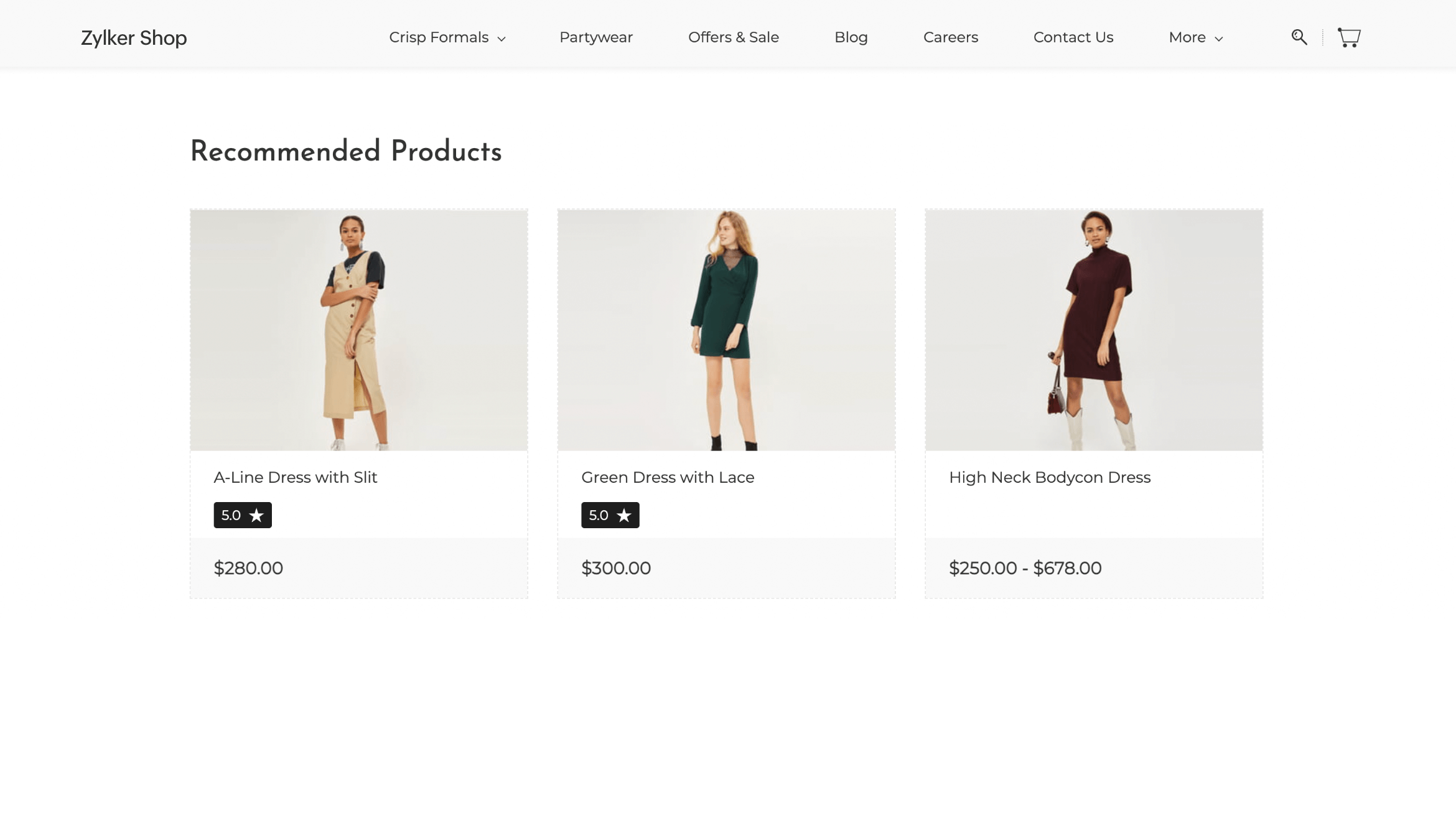Sure, here's a detailed and cleaned-up caption for the image:

---

A screenshot from the website "Gilker Shop" showcases its organized layout and product offerings. At the top, the image displays a gray border. On the left, the site name "Gilker Shop" is prominently featured, followed by a series of menu options: "Crisp," "Formals," "Just Drop Down," "Party Wear," "Offers and Sale," "Blog," "Careers," "Contact Us," "More Drop Down," along with icons for search and shopping cart positioned on the far right.

Beneath this header, the background shifts to white. In the top left corner, there's a section titled "Recommended Products," which is followed by three square-shaped images showcasing different dresses.

1. The first image features a woman wearing a tan A-Line dress with a black shirt underneath. The description "A-Line Dress with Slit" is written below the image, accompanied by a black box indicating a rating of 5.0 stars and a gray box listing the price at $280.
   
2. The next image presents a woman in a short, long-sleeve green dress with lace details. This dress is labeled as a "Green Dress with Lace," also rated at 5.0 stars (displayed within a black rectangle), priced at $300 (within a gray rectangle).
   
3. The final image captures a brown short-sleeve dress with the description "High Neck Body Con Dress." Below, a gray rectangle indicates a price range of $250 to $678.

---

This caption provides a clearer and more structured description, making it easy to visualize the webpage layout and specific product details.